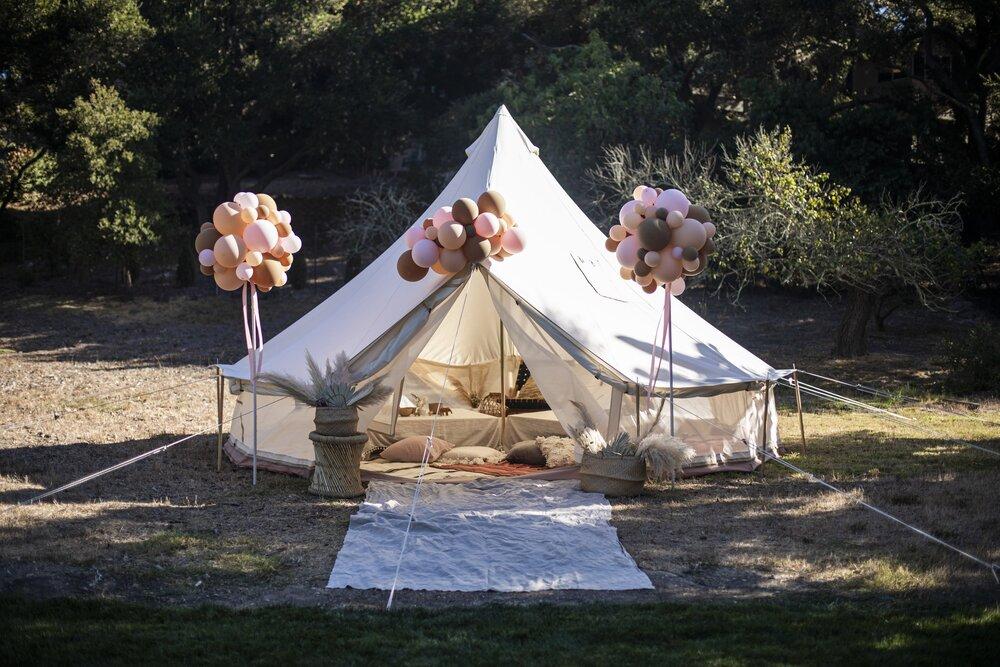In this picturesque photograph of a glamping setup, the scene is set amidst a landscape featuring both areas of dead brown grass and vibrant green patches. The location, which could either be a park or a backyard, is surrounded by tall trees, adding a serene natural backdrop. At the heart of this setup stands a strikingly elegant white tent with a high peak and gently sloping sides. The tent's entrance flaps are opened wide, offering a glimpse into a cozy interior enhanced by rich detail. 

Inside the tent, a bed adorned with an array of pillows in hues of tan, white, brown, and a hint of peach creates a welcoming and comfortable retreat. The floor is lined with soft peachy-colored carpeting, adding an additional touch of warmth. Outside the tent, sprucing up the aesthetic, are flower pots brimming with vibrant blooms, positioned on either side of the entrance. Complementing the floral decorations are bunches of balloons in shades of pink, light brown, and dark brown, festively attached to three posts. 

A charming cloth is laid out on the green grass path leading into the tent, enhancing the inviting and luxurious ambiance of this glamping experience. The overall scene captures a delightful blend of nature and comfort, making for a visually stunning and serene outdoor retreat.